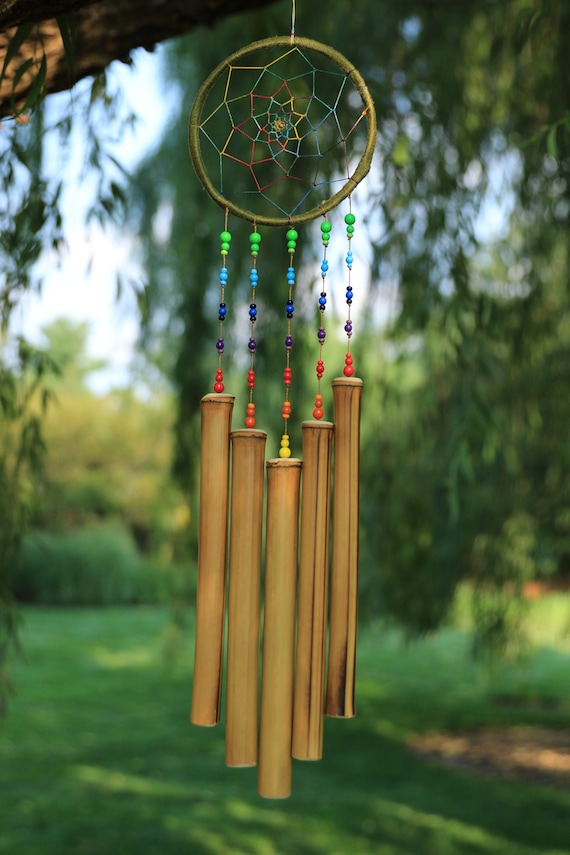This vibrant, outdoor, daytime photograph captures a dreamcatcher-style wind chime hanging from a branch with green leaves. The top part of the wind chime features a wooden circle with a colorful, spiderweb-like filigree pattern in shades of yellow, green, blue, and red, resembling a star or flower. Attached to this circle are five strings adorned with beads in various colors, including green, light blue, blue, darker blue, purple, red, orange, and yellow. These beads culminate in the suspended cylindrical bamboo pieces that serve as the chimes. The background of the image is softly blurred, revealing hints of grass at the bottom, obscured trees, and sky, highlighting the intricate and colorful details of the wind chime.